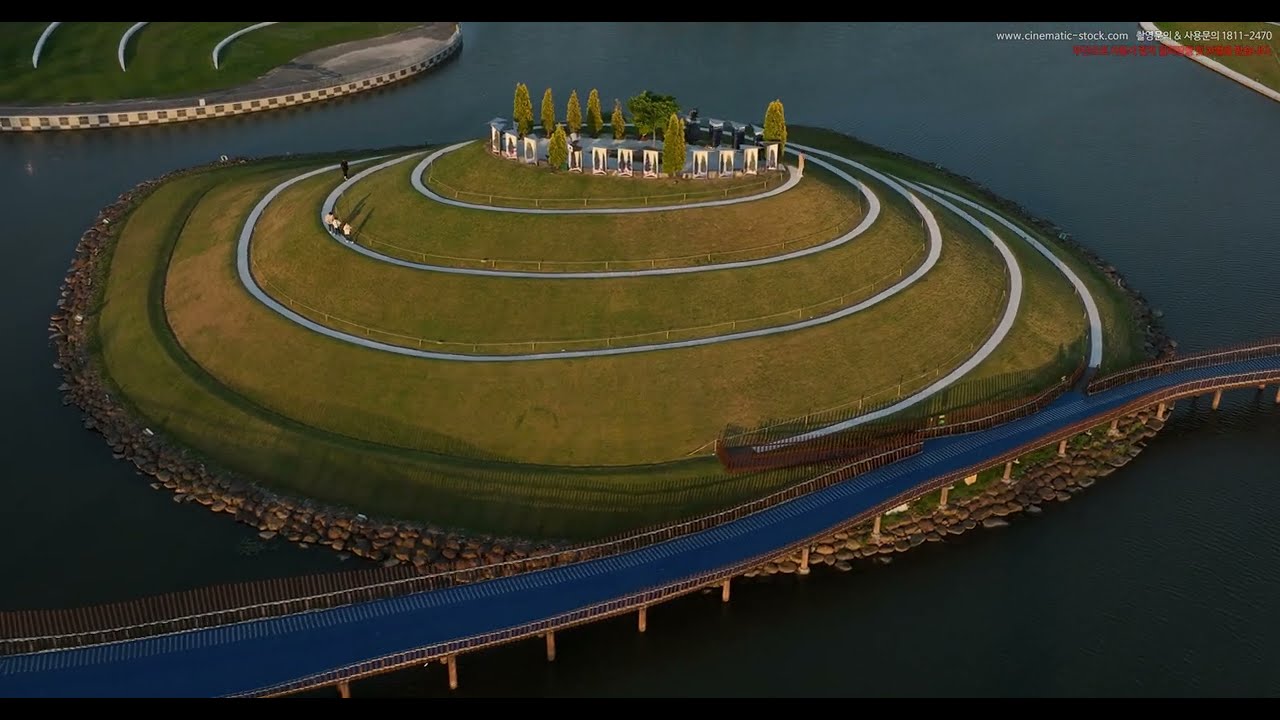In this captivating aerial image, we observe a distinct circular island set amidst a deep blue body of water, surmounted by meticulously trimmed green grass reminiscent of a golf course putting green. A prominent feature is the white, spiral pathway that ascends the island, bordered by stone walls and railings, leading to the island's peak. The path appears marked by concentric white circles, which create a visually striking pattern as they spiral upwards. At the summit, a cluster of rectangular, stone structures and a few tall, narrow trees stand out, adding an architectural element to the landscape. Numerous tiny figures can be seen traversing this winding path, enhancing the sense of scale and activity. To the bottom right of the image, a roadway begins at the lower left corner, crosses mid-center, and stretches to the far right, partially hidden by the terrain. Additional grassy mounds with similar features are visible in the upper left corner, further punctuating the scene. Small, discernible text with “WWW” and red lettering appears to the right, likely identifying the source of the image. The island's orderly and symmetrical construction suggests it may be a man-made structure, designed with aesthetic and recreational purposes in mind.